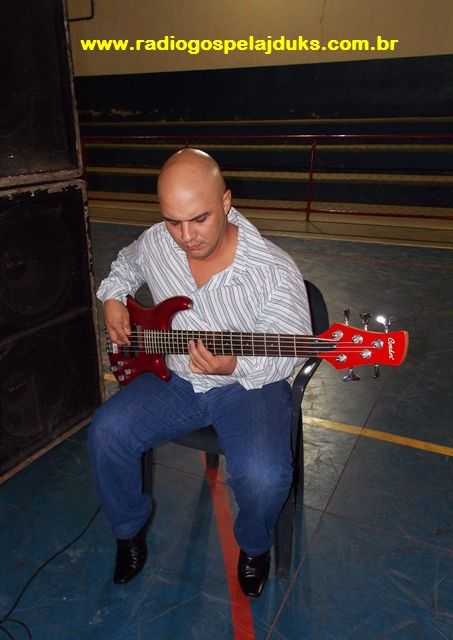In this detailed photograph, a bald man with a Hispanic appearance sits in a black plastic chair, deeply focused on playing a red electric guitar that rests on his right leg. His attire includes a white shirt with vertical gray and blue stripes, blue jeans, and black leather shoes. His shirt is unbuttoned at the collar, revealing a glimpse of his chest. The setting appears to be indoors, possibly a gymnasium or a train station, given the blue rubber floor beneath him, which is scuffed and features red and yellow lines.

Behind him, a white wall transitions into a dark blue section adorned with horizontal yellow lines. In front of this wall stands a distinct fence composed of red vertical and horizontal bars filled with black chain-link mesh. Prominently displayed on the fence is the URL "www.radiogospeladdukes.com.br" in white letters. To the left of the man, two large grey speakers, each with three visible circles on the front, are stacked on top of each other. A thin black wire snakes across the floor near the speakers, indicating the electric guitar is plugged in but out of the frame. The man remains absorbed in his music, fingers deftly moving along the neck of the guitar.